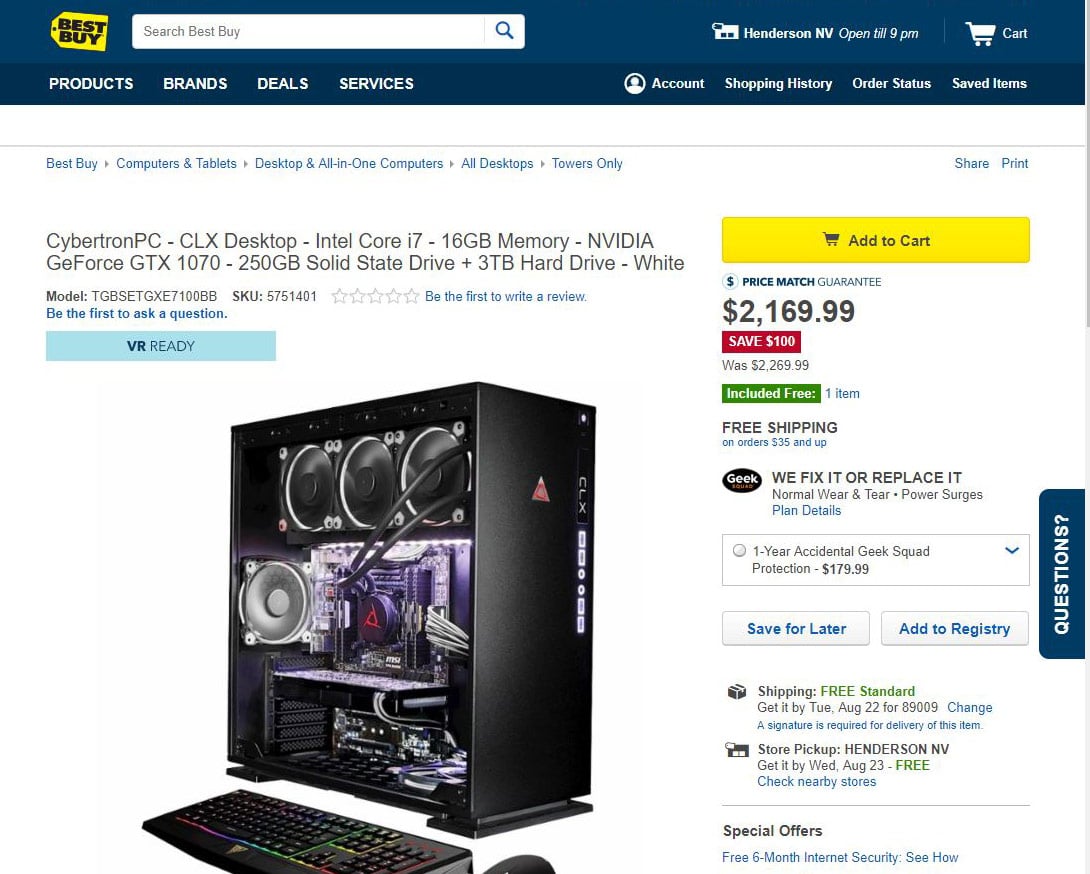The top of the webpage displays the iconic yellow Best Buy tag with "Best Buy" written in bold black letters, and directly below it is a blue search bar labeled "Search Best Buy." The webpage also indicates that the store in Henderson, Nevada is open until 9 p.m., alongside a notification that the shopping cart is empty. Navigational options are listed in white font and include categories like Products, Brands, Deals, Service, Account, Shopping History, Order Status, and Saved Items.

The focus of the page is a featured product: the Cybertron PC CLX Desktop. This high-performance desktop is detailed with specifications such as an Intel Core i7 processor, 16GB of memory, an NVIDIA GeForce GTX 1070 graphics card, a 250GB solid-state drive, and a 3TB hard drive. It is a white model identified with the code TGBSETGXE707100BB.

Accompanied by a striking image, the desktop is showcased with its side panel open, revealing purple LED lights and cooling fans — three or possibly four — ensuring efficient thermal management. The listed price of the desktop is $2,169.99, marked down from its original price of $2,269.99, offering a $100 saving. The product also benefits from Best Buy's price match guarantee and includes a promotion for free shipping on orders over $35.

Additional options highlight Geek Squad protection plans, covering accidental damage and power surges for one year at an extra cost of $179.99. Customers are invited to write a review or ask questions about the product, identified by SKU 5751401. The options to add the item to the cart, save for later, or add it to a registry are prominently displayed.